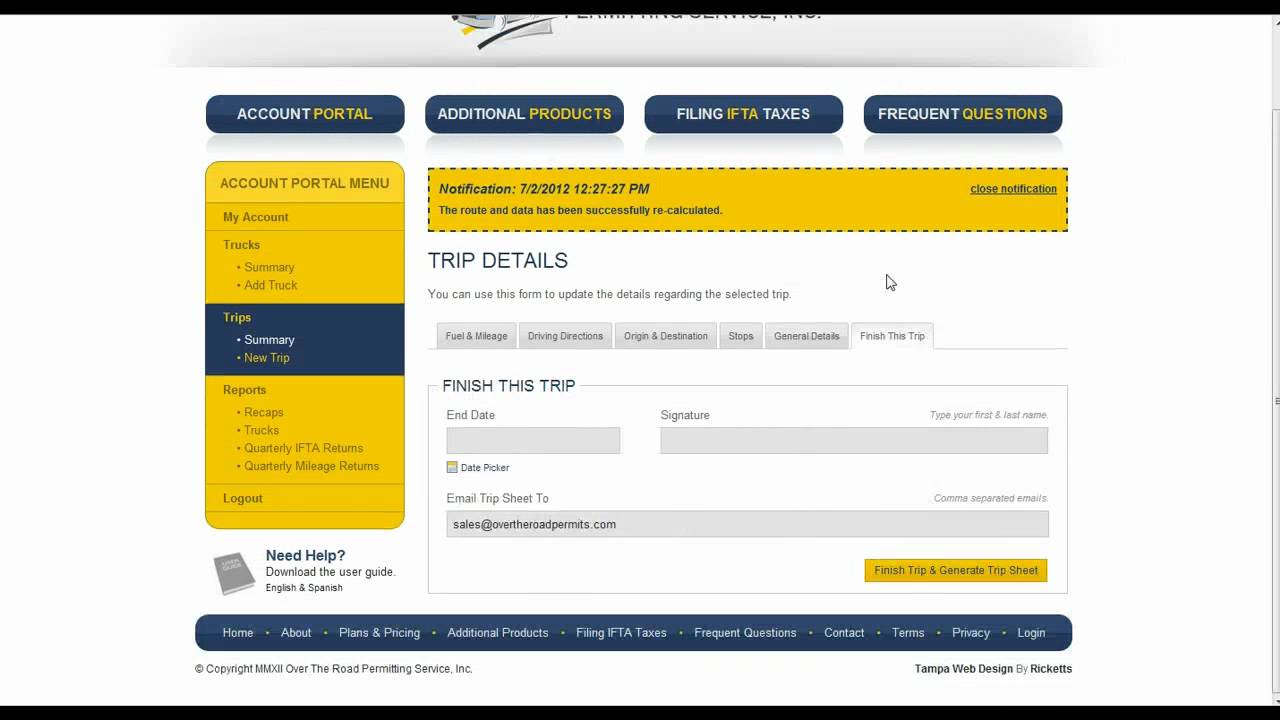This is a detailed screenshot of a trip booking website with a predominantly white background. The top features a gradient light gray header containing partially visible, unreadable text. Directly beneath this header, four dark blue rectangular sections with rounded corners are laid out horizontally. Each section contains text with distinctive color patterns: 

1. "Account Portal" with "Account" in white and "Portal" in yellow.
2. "Additional Products" with "Additional" in white and "Products" in yellow.
3. "Receiving IFTA Taxes" with "Filing" and "Taxes" in white, while "IFTA" is in yellow.
4. "Frequent Questions" with "Frequent" in white and "Questions" in yellow.

Below these rectangles is a mustard yellow box edged with a dotted black outline, displaying the notification "7-2-2012-1227-27pm. The route and data has been successfully recalculated. Close notification" – the latter being underlined in the top-right corner.

Further down, the title "Trip Details" is presented alongside instructions indicating that users can use the form below to update trip details. Six tabs are listed beneath this title, with the first five in light gray: "Fuel and Mileage," "Driving Directions," "Origin and Destination," "Shops," and "General Details." The sixth tab, highlighted in white, is labeled "Finish This Trip," and is currently selected. 

Following these tabs, a light gray box labeled "Finish This Trip" is displayed. It contains fields titled "End Date" and "Signature," each represented by a blank light gray box. Below the "Signature" field, italic text prompts users to "type your first and last name." Another section labeled "Email Trip Sheet To" includes a light gray box pre-filled with "sales@overtheroadpermits.com" and notes that comma-separated emails can be entered.

At the bottom, yet another mustard yellow box prompts users with "Finish Trip and Generate Trip Sheet." To the left of the entire layout, there is a vertically oriented mustard yellow menu.